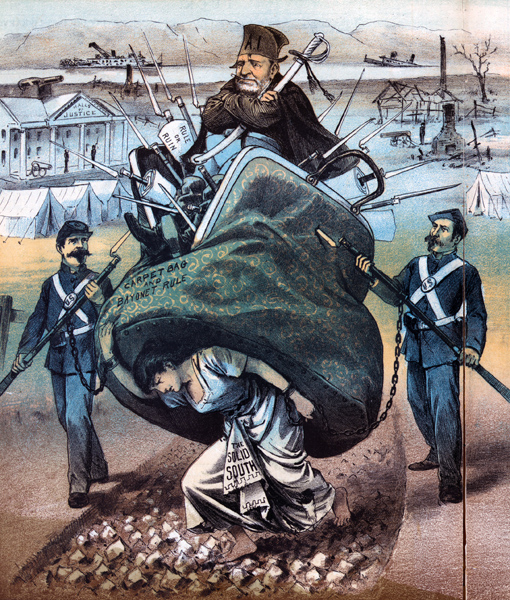This is a detailed political cartoon depicting a lobo man seated atop an oversized coin purse, surrounded by numerous sharp, pointy weapons with white blades and black handles. The lobo wears a black towel hat and a black cap. A sign to his left reads "RULE OR RUIN," and the purse itself is labeled "CARPET-BAG AND BAYONET RULE." Below, a woman chained to a military man is carrying the large purse on her back, with her dress bearing the phrase "SOLID SOUTH." Flanking the purse on either side are two U.S. soldiers in military uniforms, each armed with long guns and decorated with crossbands inscribed with "US." One soldier appears to be piercing the purse with his gun. In the background looms the "Hall of Justice," adding to the heavily metaphorical and satirical nature of the illustration.